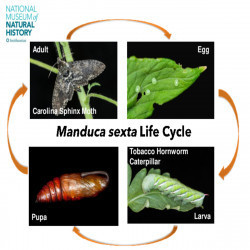The image is an educational illustration titled "Manduca Sexta Life Cycle," and it is credited to the "National Museum of Natural History," the latter being written in blue text at the top left corner. The illustration is organized into a 2x2 grid, showcasing the life stages of the organism. Each of the four rectangular photographs is set against a black background with accompanying text and visual elements. The top left image shows an adult moth perched on a green plant stem, labeled "Adult." The top right image depicts a green leaf with small, white oval eggs labeled "Egg." The bottom right image features a green caterpillar-like larva on a leaf, labeled "Larva." Lastly, the bottom left image presents a brownish-orange pupa, labeled "Pupa." Orange arrows connect each image in a clockwise sequence, visually indicating the cycle from one stage to the next. In the white space between the two rows, the phrase "Manduca Sexta Life Cycle" is written in black text.